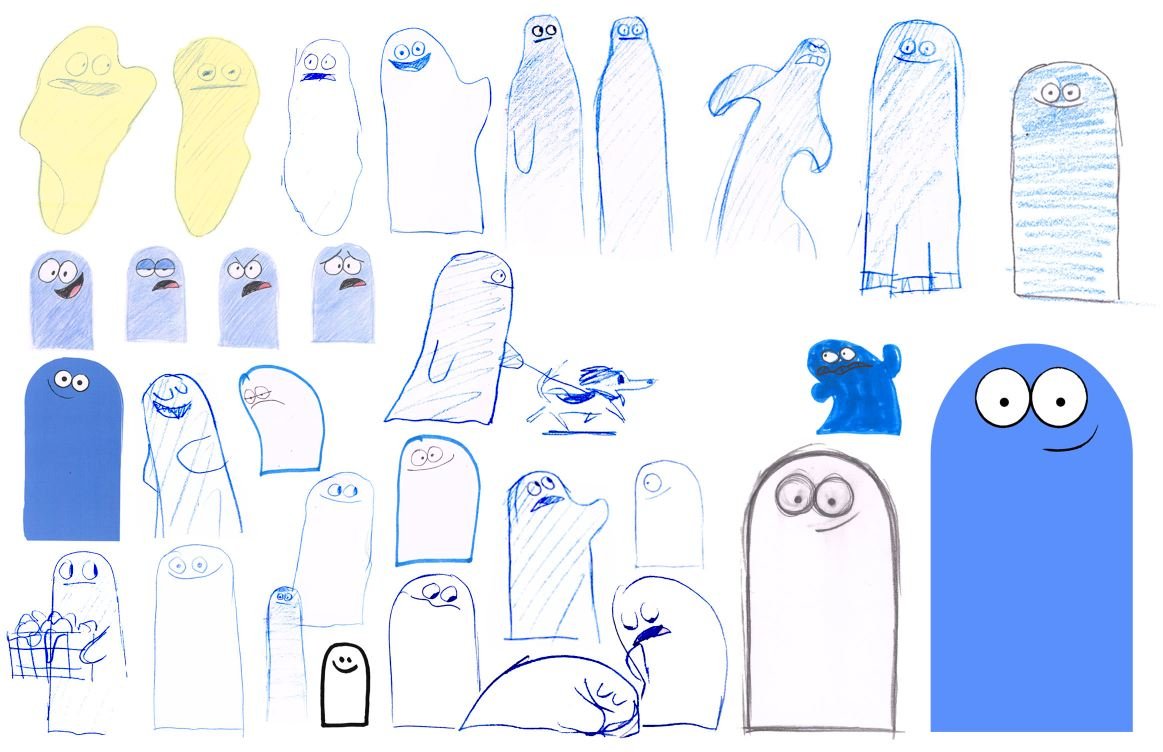This artwork depicts a series of cartoonish ghost sketches on a white background in a landscape orientation. The ghosts are represented in various renditions, with the majority outlined or shaded lightly in blue. In the upper left corner, two sketches stand out with a light yellow shading, while a few in the upper right corner are shaded in blue. The ghosts are presented in different states and moods: some are laughing and appear silly, while others try to evoke a scarier vibe. Notably, one ghost is walking a dog, and another is lying down with a distressed ghost looking over. There are also four smaller ghosts akin to press-on nails, each adorned with a cartoony face. The most detailed ghost is in the bottom right corner, resembling a tombstone with large white eyes and an off-center smile. Overall, this image seems to be an artist's exploration of a ghost character in different scenarios, potentially for a cartoon strip.